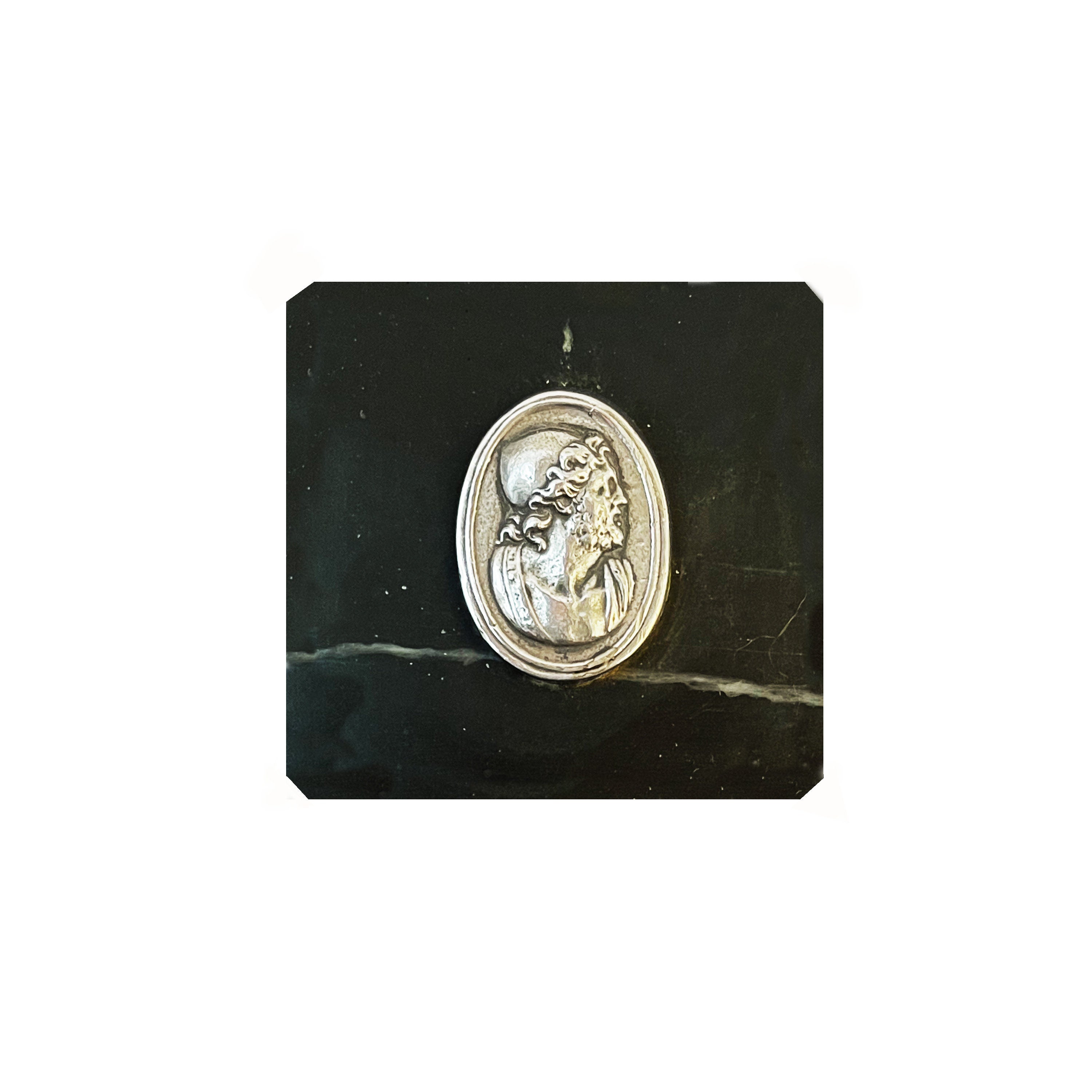This photograph captures an antique pewter or silver oval pendant, displayed on a striking black marble surface with a distinctive greenish vein running horizontally about a quarter way down. The pendant prominently features an intricately engraved bust of a man in ancient attire, presumed to be either Roman or Greek, given his flowing wavy hair, slight beard, and cone-shaped hat that somewhat resembles an octopus body. His side profile, facing right, showcases his detailed facial features as well as a portion of his chest and shoulders, clad in a traditional robe. The pendant is elegantly bordered with a raised trim, enhancing its historical and artistic significance. The overall scene is framed with the pendant's lustrous surface contrasting against the deep, patterned marble backdrop, accentuating the artifact’s timeless charm and craftsmanship.